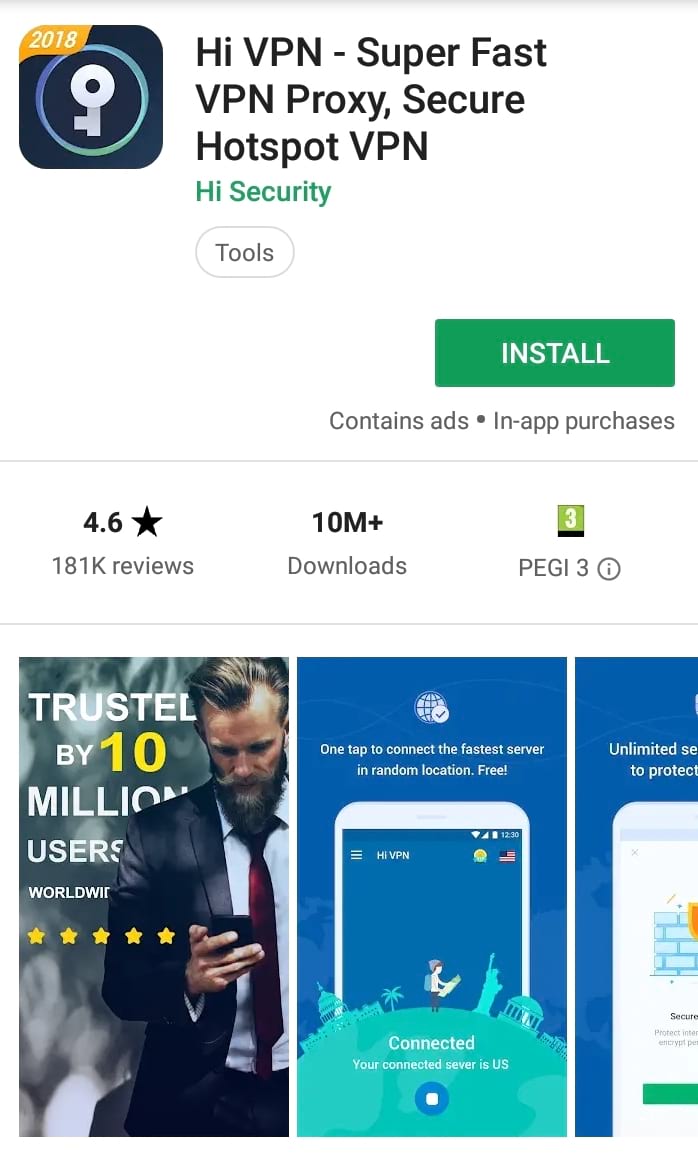This image is a detailed screenshot of a Google Play website page showcasing an application. The design appears with a clean white background.

- In the top left, there is a prominent dark blue square icon featuring a light blue circle within it. Inside the circle, a downward-facing key icon is visible. A small orange flag with "2018" written on it is positioned at the top left corner of the blue square.

- To the right of this icon, the application's name is displayed: "HiVPN-Superfast". Below this, three lines describe its functions: "VPN Proxy Secure" and "Hotspot VPN", both in black text. The developer's name "HiSecurity" is presented beneath in smaller green font. Additionally, there's a white, sideways oval button marked "Tools" in black text.

- Further down on the right side of the page, a prominent green rectangular button labeled "Install" in white is visible. Directly below this, in smaller font, it mentions "Contains ads • In-app purchases".

- Continuing downward, key statistics are displayed: a 4.6-star rating, over 10 million downloads, and a PEGI 3 rating, each accompanied by its corresponding icon.

- The lower section of the screenshot then features a few vertical ads, seen sliced or vertically aligned, adding to the overall informational layout of the page.